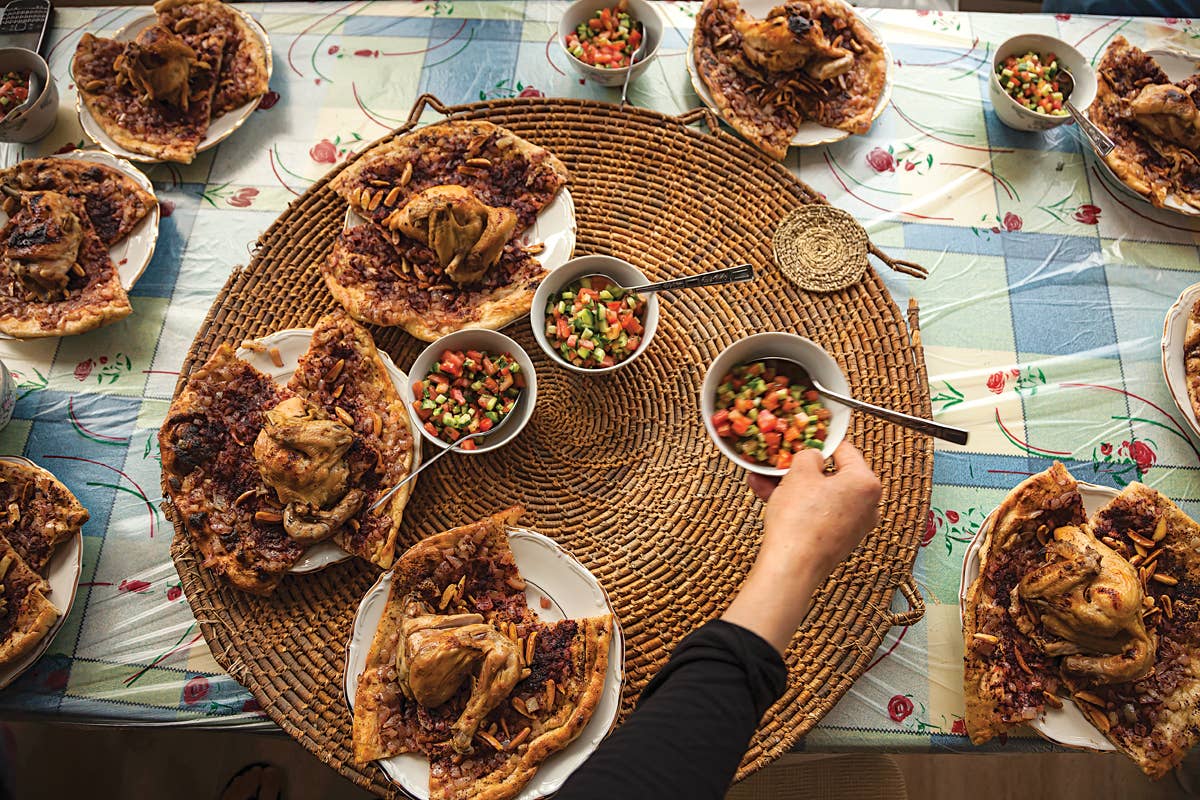This is an overhead view of a vibrant meal spread out on a table adorned with a wide plaid tablecloth featuring green, pale yellow, light blue hues, and red flowers. At the center of the table is a large circular rattan serving tray, woven from reeds, accented by smaller coasters or serving mats placed on top. Surrounding the tray are multiple dishes, including three plates with diced vegetables, possibly salsa or beans, each with a silver spoon. Centered on the tablecloth are 10 plates, each holding a half chicken that appears to be pan-fried, resting on flatbread. The flatbread is topped with a sumac-onion mixture, hinting at a dish similar to moussakaan. Additionally, some plates also feature a cucumber and tomato salad. The arm of a person is visible at the bottom of the photo, implying the image was captured from an overhead perspective.